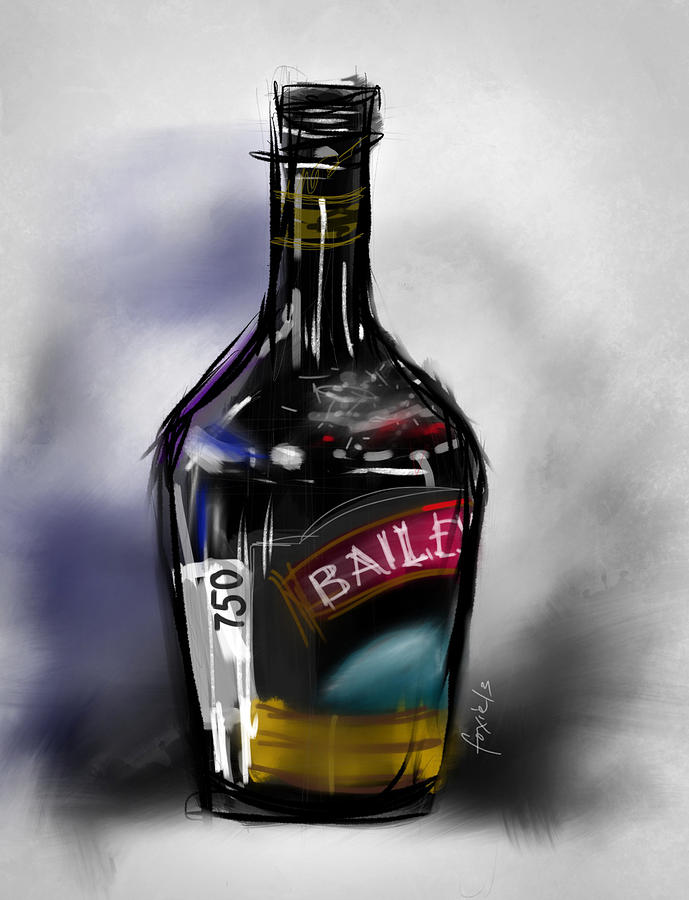This image is an abstract, hand-drawn painting of a 750ml bottle of Bailey's Irish Cream. The bottle is depicted in a cartoonish, iconic style, featuring a black color with a label that has the brand name "Bailey's" written in white letters on a maroon background. Below the label, there's a yellow section with a teal, odd-shaped circle, and further down the bottle, there's a white sidebar detailing the size. The artist's signature, which appears to read "Fox Eels," is written in a white script font along the side. The background consists of varying shades of grey and black, with smudges creating a shadowy effect to highlight the bottle. The overall setting has white and grey lines and streaks running up to the neck of the bottle, adding a textured depth to the composition. The bottle sits against a background that transitions from darker shades in the center to lighter greys, giving a sense of depth and focus to the subject.